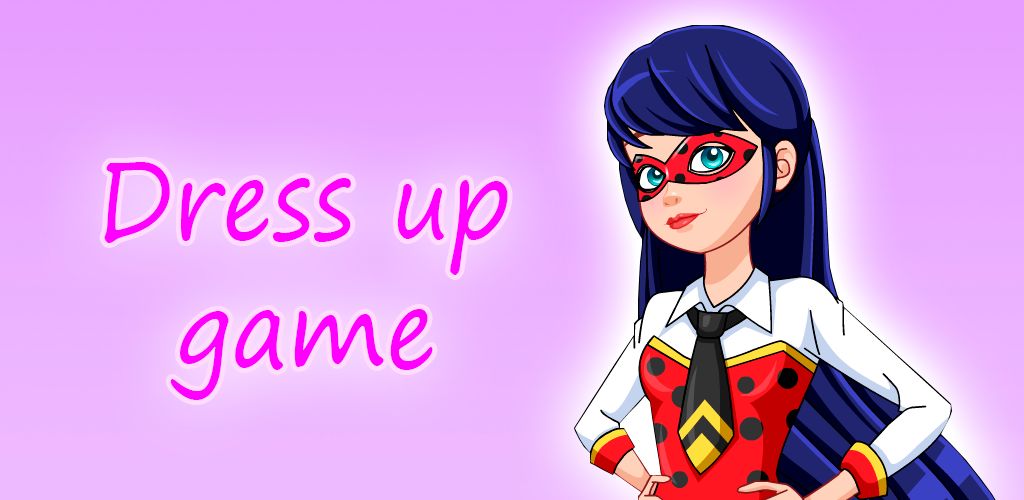The banner advertises a "Dress Up Game" against a light pink background, with the text "dress up game" in darker pink letters bordered by white on the left side. On the right, a cartoonish woman, visible from the waist up, strikes a confident pose with her hands on her hips. She dons a red corset with black polka dots over a white button-up collared shirt, complemented by a black tie with yellow stripes. Her very long black hair cascades down her back, resembling a cape, and she wears a matching red mask with black dots over her eyes, which are blue and focused forward while her body angles towards the left corner. The overall style is reminiscent of computer-generated or hand-drawn anime graphics, incorporating colors like pink, tannish peach, red, black, blue, and white. Her vivid appearance, almost glowing against the light background, emphasizes a playful and heroic cosplay theme.